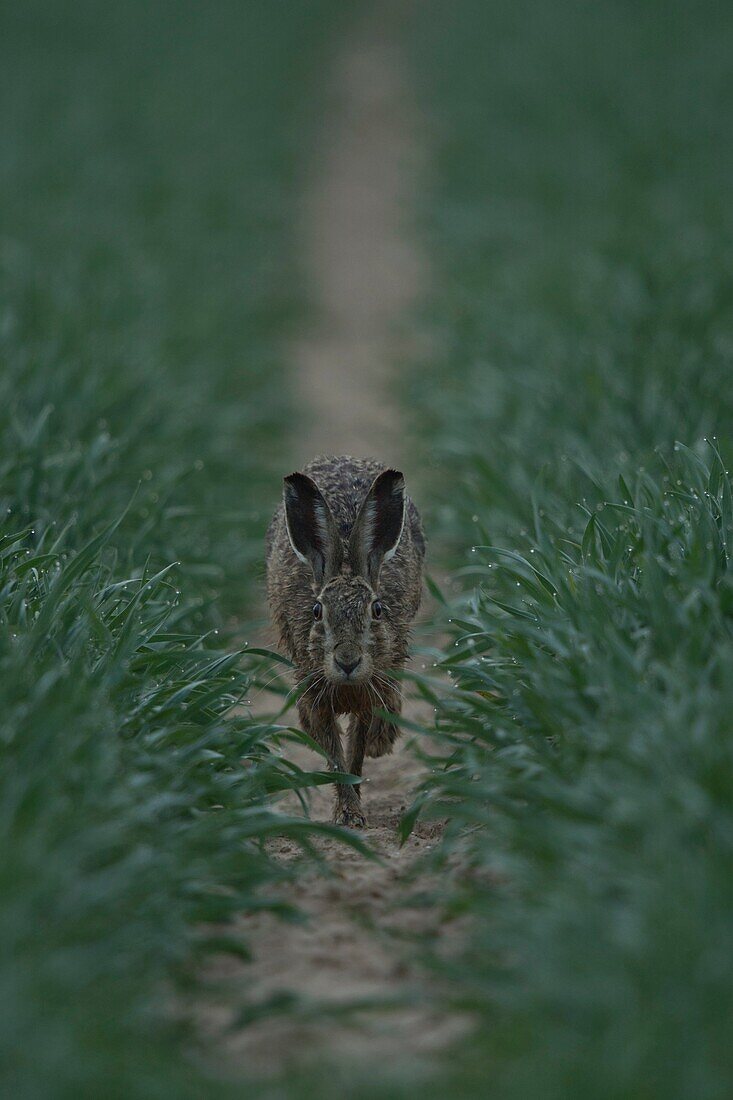This detailed portrait-shaped photograph captures a dynamic moment in nature, featuring a jackrabbit in mid-motion as it hops directly towards the viewer along a narrow, light brown dirt path that extends from the front to the back of the image. This path is flanked on both sides by taller grass, which displays individual blades and dew drops, especially in the foreground. The jackrabbit's fur reveals a nuanced mix of brown, white, and mottled gray, with distinctively tall ears that are dark brown at the tops and light brown towards the middle. The photograph, with its sharp focus on the jackrabbit and the immediate surroundings, shows the animal’s large, detailed eyes, prominent whiskers, and extended legs. The background and the extreme foreground are artistically blurred, drawing attention to the rabbit as the focal point and enhancing the sense of motion against the blurred, green-hued grass behind it.